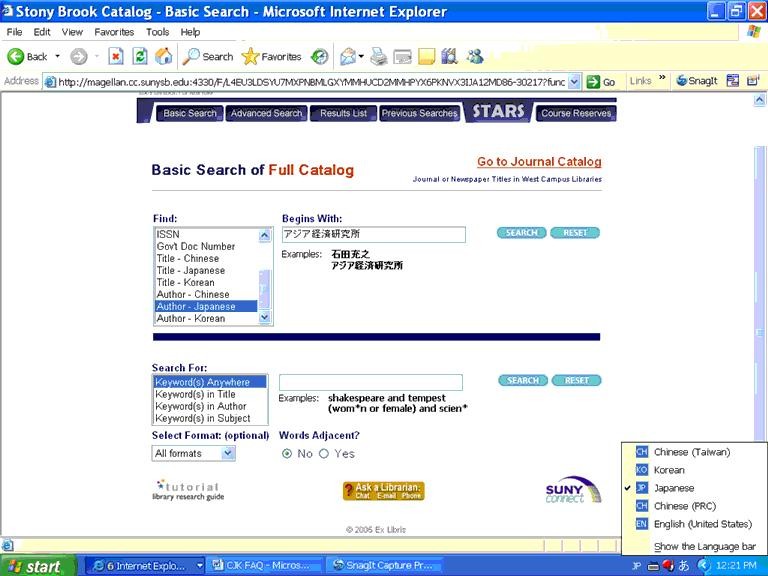The image depicts an old web page interface from the era when Windows XP or Windows Vista was prevalent. At the very top of the screen, there is the Internet Explorer symbol on the top-left corner, alongside text that reads "Stony Brook Catalog - Basic Search - Microsoft Internet Explorer" in bold white lettering. Below this, there is a beige-colored menu bar with options: 'File,' 'Edit,' 'View,' 'Favorites,' 'Tools,' and 'Help.'

A light gray line divider separates this menu from the navigation bar below. The navigation bar features several options starting with a green circular 'Back' button with a white left-pointing arrow and black text that reads "Back." Next to it, there is a downward arrow indicating more options. Following this is a grayed-out 'Forward' button with a right-pointing arrow, which is currently disabled. Then, there is a red 'X' on a white background for stopping the page load, followed by a green 'Refresh' symbol on a white background for refreshing the page. Adjacent to these icons is a house symbol, indicating the home page, separated by another light gray divider.

Further along the navigation bar are a series of icons: a magnifying glass labeled "Search," a star symbol for "Favorites," and a clock symbol. Another light gray divider follows before an envelope with a downward arrow (likely for mail or downloads), a printer symbol for printing the page, a writing pad or post-it note, and icons representing a library or book search. The final icon in this series is the MSN logo.

The main content area of the webpage starts with a blue menu bar that gradually transitions to a purple hue. This bar includes options such as "Basic Search," "Advanced Search," "Results List," and "Previous Searches." Below this menu, in large bold letters, the term "STARS" is prominently displayed, followed by "Course Reserves" in the same font style. The phrase "Basic Search of" appears in navy blue text, succeeded by "Full Catalog" in bright orange text.